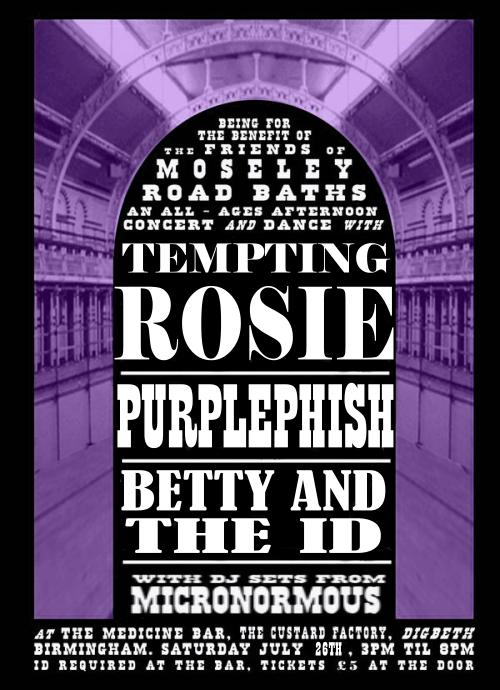The image depicts a poster advertisement for an all-ages afternoon concert and dance event. The poster features a distinctive and visually striking design with a purple-hued archway background that resembles the interior of a building, possibly with barred windows on either side, giving an almost ethereal glow. A central black arched frame contains bold, capitalized white text detailing the event. The headline reads "Being for the Benefit of the Friends of Moseley Road Baths." Performing acts include Tempting Rosie, Purple Fish, Betty and the Id, complemented by DJ sets from Micronormous. The event is scheduled to take place at the Medicine Bar, located in the Custard Factory in Digbeth, Birmingham, on Saturday, July 26, from 3 p.m. till 8 p.m. Entry requires ID, and tickets are priced at £5, available at the door.